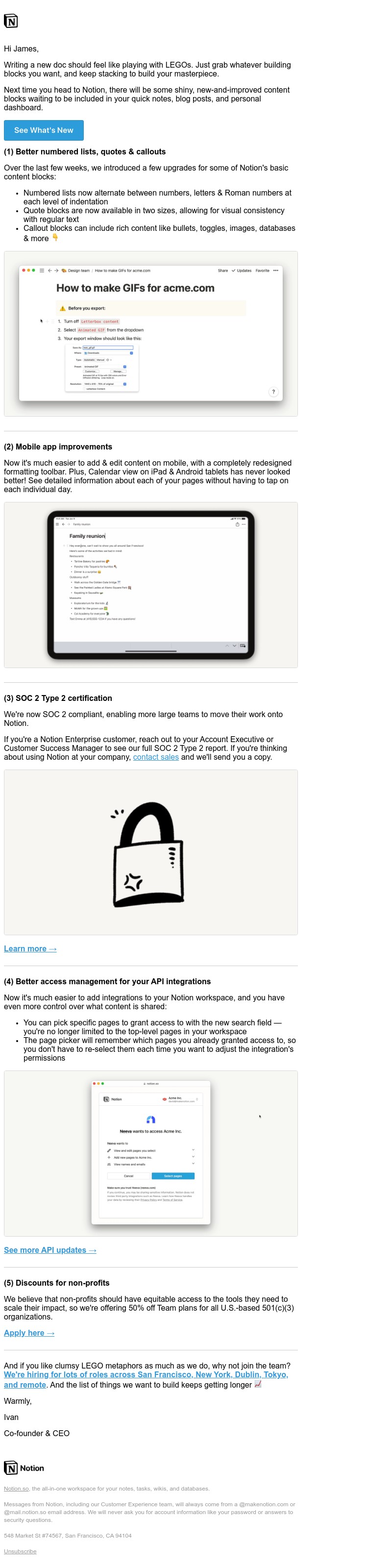Image Caption: 

This screen capture, taken from a digital device, displays a set of instructions. The blurred text is difficult to read but outlines a step-by-step guide on creating GIFs for Acme.com. At the top, an introduction appears, followed by detailed instructions accompanied by various diagrams. The first diagram features a rectangular window with a white background, prominently displaying the text "How to Make GIFs" in black. The subsequent images are less clear but provide further illustrative guidance. The third image resembles a large rectangular padlock with a black curved lock at the top. The fourth image, also set against a white background, includes a smaller rectangular section with some blue inscriptions, although the exact details are hard to decipher.